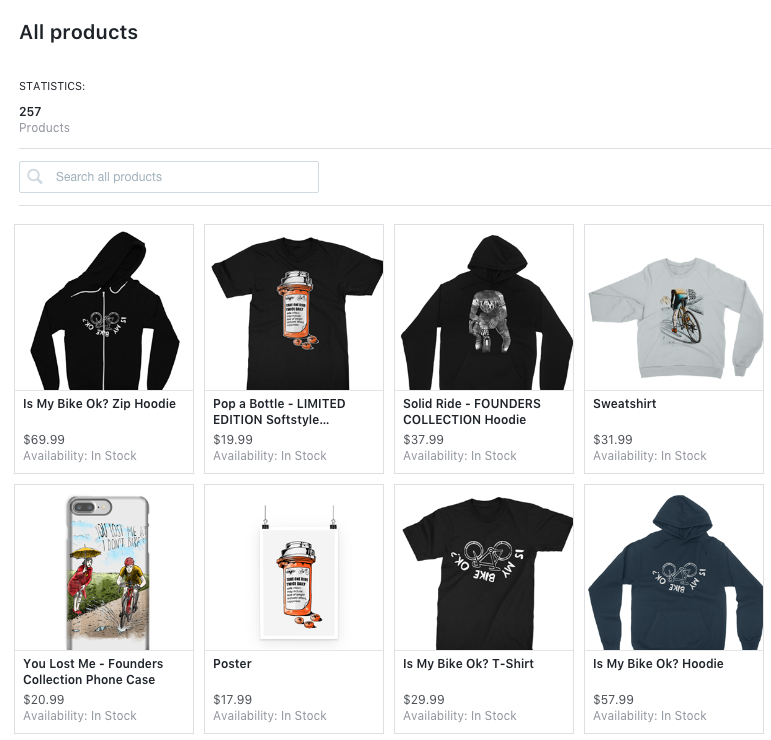The image is a cropped screenshot of the "All Products" section on a website, focusing on the first two rows of products. The header and other options are edited out, leaving a clear view of the essential elements. At the top left, bold black text reads "All Products," followed by "Statistics:" and "257 products," with "257" also in bold black font. Just below this information is a search bar labeled "Search All Products."

The products are displayed in two horizontal rows of four thumbnails each. The first product in the top row is a hoodie titled "Is My Bike OK? Zip Hoodie." The price and availability details are located at the bottom left of the thumbnail. The second product is a t-shirt, presented as a flat lay mock-up, titled "Pop A Bottle Limited Edition," with its price and availability also positioned at the bottom left. The remaining products follow the same format: a thumbnail image, the product title below it, and the price and availability details at the bottom left.